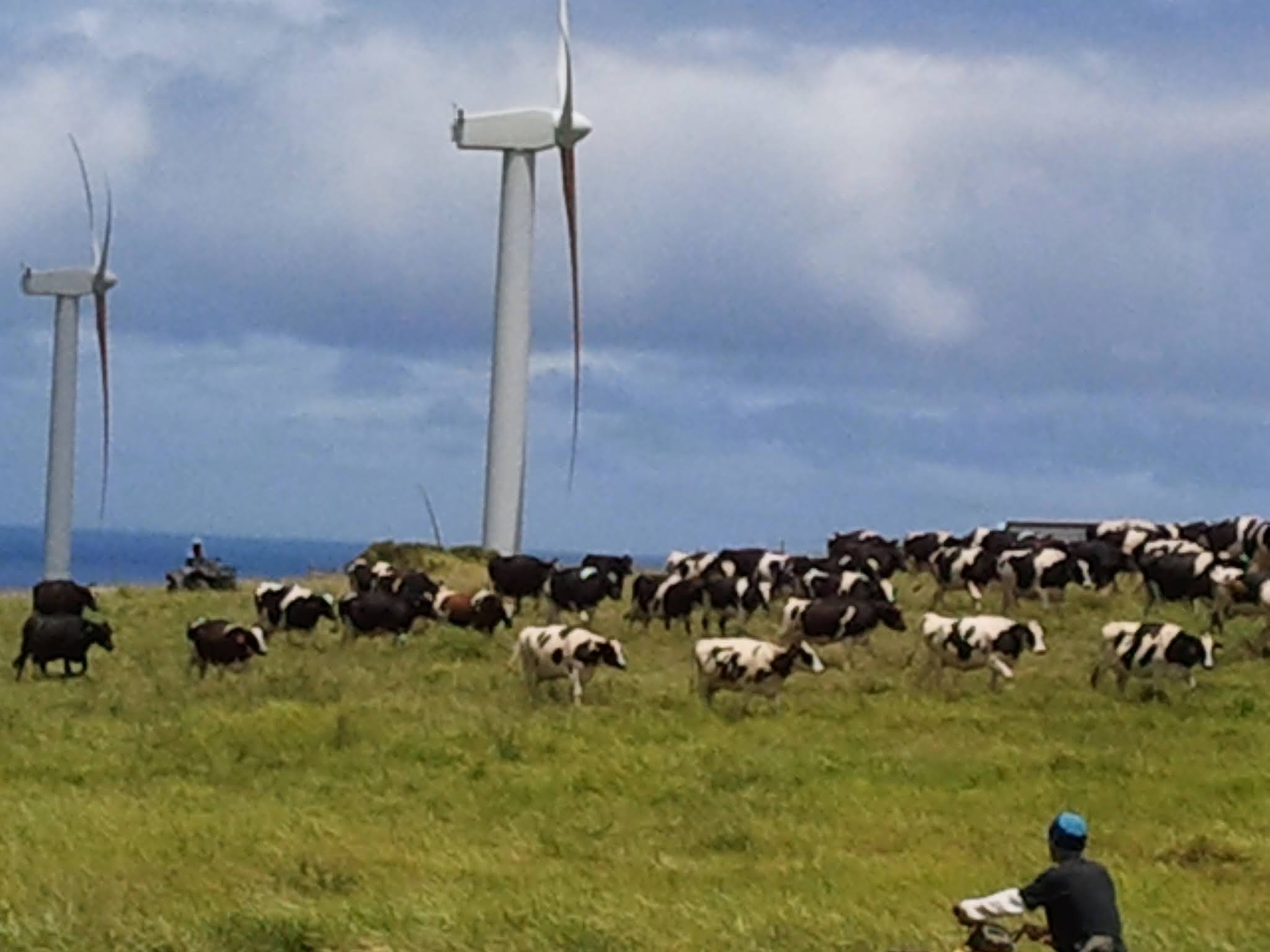The photograph depicts a modern coastal farm featuring a lush, grassy green field filled with black and white dairy cows, suggesting it was taken in summer. In the foreground, at the bottom right, there is a farmer wearing a blue hat and black shirt with white sleeves, partially visible as he rides a quad bike. Both farmers are using these vehicles to wrangle the herd of large, healthy cows, which are moving toward the right side of the image. To the left, another farmer on an ATV can be seen in the background. Dominating the scene are two large, white wind turbines, signifying the farm's modernity. A thin sliver of deep blue sea is visible in the far background, confirming the coastal setting. The sky above is densely packed with thick clouds, casting a dim light over the vivid green landscape.